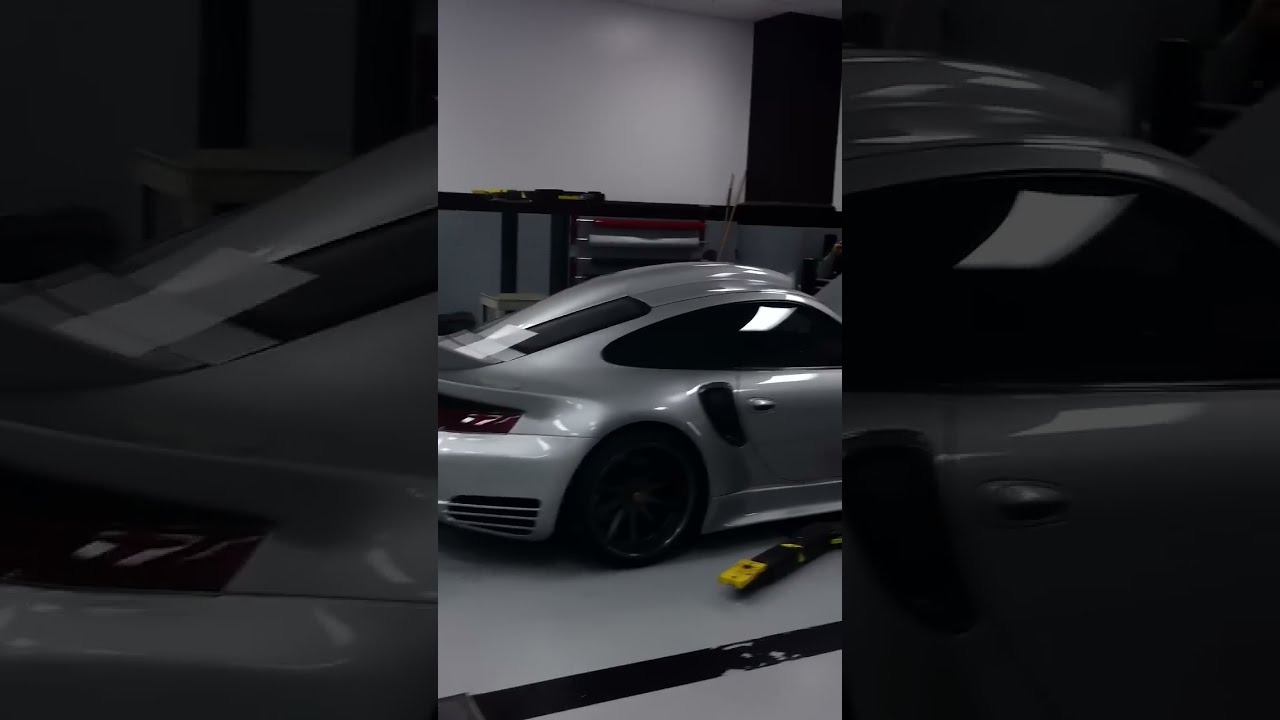This image is a blurry, out-of-focus, low-quality photograph of the rear of a high-end, light silver sports car. The image captures a candid scene, likely taken in an enclosed environment such as a car dealership showroom or a car show. The car, which exhibits a futuristic and innovative design with notable black trim, is centrally positioned within the frame. Despite the blurriness, the license plates are present though unreadable. Two individuals, dressed in black clothing, stand on either side of the car, and in the background, other vehicles, including a red car, can be vaguely seen. Vertical black bars, around two inches wide, run along each side of the image, suggesting it might be taken through a window or framed in some manner. The full picture measures approximately eight inches wide by four to five inches tall, lacking any text or website listings, making it evident that this is an amateur, spontaneous capture. The entire background is out of focus, highlighting the stationary setting in which the car is displayed.